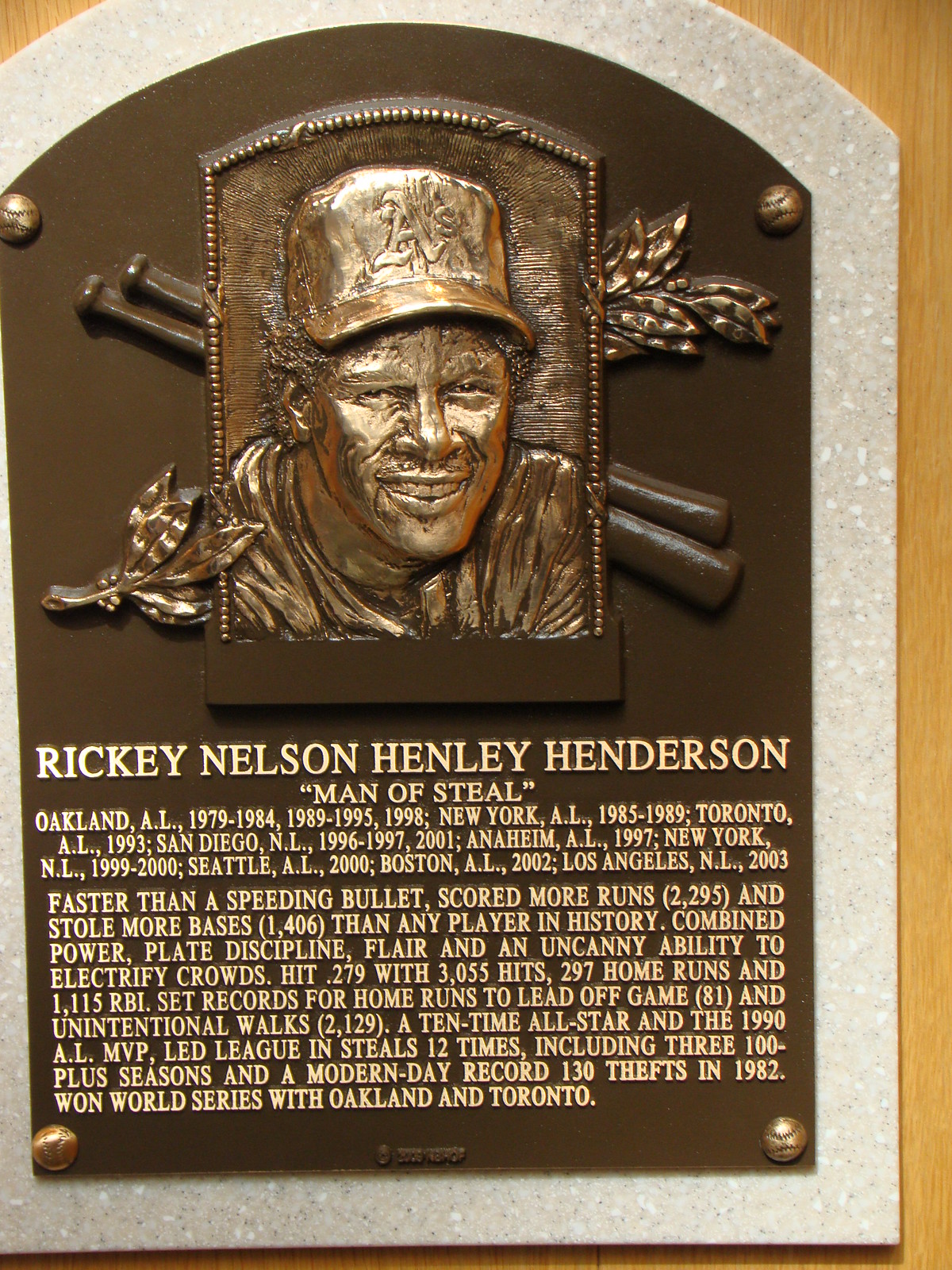This detailed Hall of Fame plaque commemorates the legendary baseball career of Ricky Henderson. The plaque is bronze and affixed to a thin, marble-like sheet, mounted on a light wooden wall with screws shaped like baseballs at each corner. It features an artistic rendering of Henderson, smiling and wearing an Oakland A's cap, against a backdrop of crossed baseball bats and a plant sprig. The plaque is titled "Ricky Nelson Henley Henderson," with the moniker "Man of Steel" prominently displayed.

The text on the plaque meticulously details Henderson's career, noting his stints with various teams: Oakland A.L. (1979-84, 1989-95, 1998), New York A.L. (1985-89), Toronto A.L. (1993), San Diego N.L. (1996-97, 2001), Anaheim A.L. (1997), New York N.L. (1999-2000), Seattle A.L. (2000), Boston A.L. (2002), and Los Angeles N.L. (2003). 

Henderson is celebrated for his remarkable achievements: scoring 2,295 runs and stealing 1,406 bases, more than any player in history. His career statistics include a .279 batting average, 3,055 hits, 297 home runs, and 1,115 RBIs. The plaque highlights his unique combination of power, plate discipline, flair, and ability to electrify crowds. Henderson set records for home runs to lead off games (81) and unintentional walks (2,129), was a 10-time All-Star, and the 1990 AL MVP. He led the league in steals 12 times, including three seasons with over 100 steals, and set a modern-day record with 130 thefts in 1982. Henderson also won World Series titles with Oakland and Toronto.